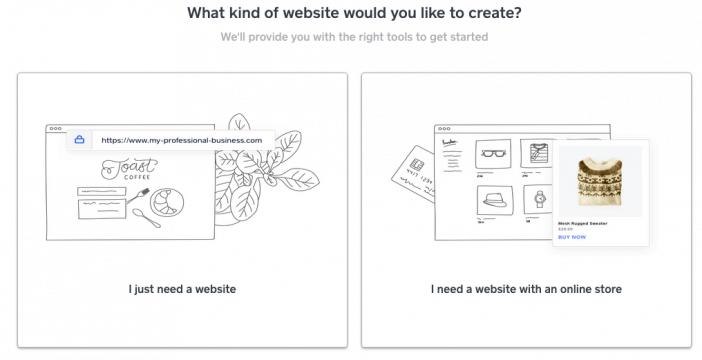Screenshot of a Web Page Creation Site:

At the center of the webpage, prominently displayed in black or gray text, is the question: "What kind of website would you like to create? We'll provide you with the right tools to get started."

Beneath this question, the page is divided into two sections:

1. **Left Side - Personal Website**:
    - Header: A recommendation from "myprofessionalbusiness.com."
    - Sample Text: "I just need a website."
    - Example: A thumbnail image of a website labeled "Toast Coffee" that features a croissant and some plants to the side.

2. **Right Side - E-commerce Website**:
    - Header: "I need a website with an online store."
    - Description: Provides tools to set up an online store to sell products.
    - Visuals: Includes images of various products such as glasses, watches, and shirts. One of the shirts has a "Buy Now" button in blue lettering.

The background beyond these descriptive boxes is blank white, without any additional elements such as a URL bar or browser interface. This likely indicates a basic starting or drop page for the web page creation site.